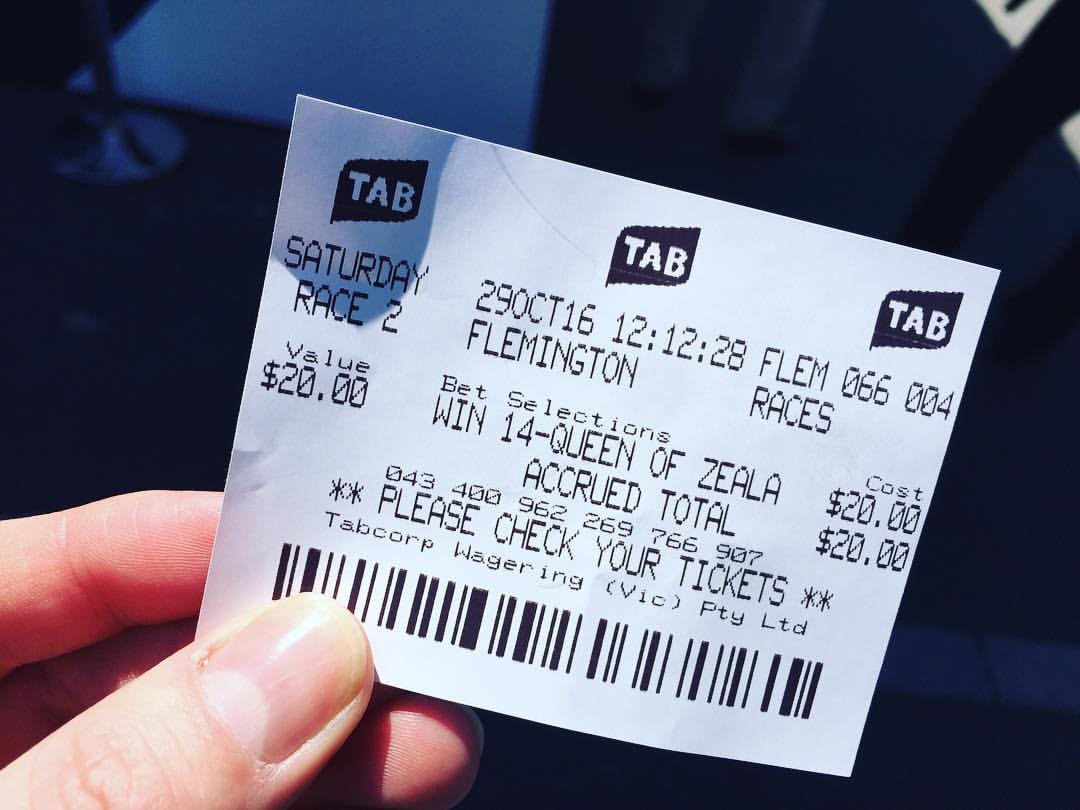In this detailed photograph, a person's hand is prominently featured holding a white ticket stub angled diagonally in the frame, with the top facing the top left and the bottom right corner. The background is a blend of navy blue, light blue, darker blue, and white, appearing as a blurred, natural light scene, likely taken outdoors during the day due to the shadows present. The ticket, primarily white with black text, is adorned with three TAB logos at the top. Below the logos, the stub features essential race details, including "Saturday, 29th October, 16:12:12" and "Race 2" at Flemington Races. The ticket specifies a bet selection for "Win, 14, Queen of Zila," with a value and cost of $20. The stub also includes a barcode at the bottom, and various wagering details, instructing to "please check your tickets," and a footer reading "TAB Corp Wagering, Vick, PTY, LTD." The photograph, in landscape orientation and showcasing realistic representationalism, emphasizes the contrast between the crisp details of the ticket and the blurred, gradient background.